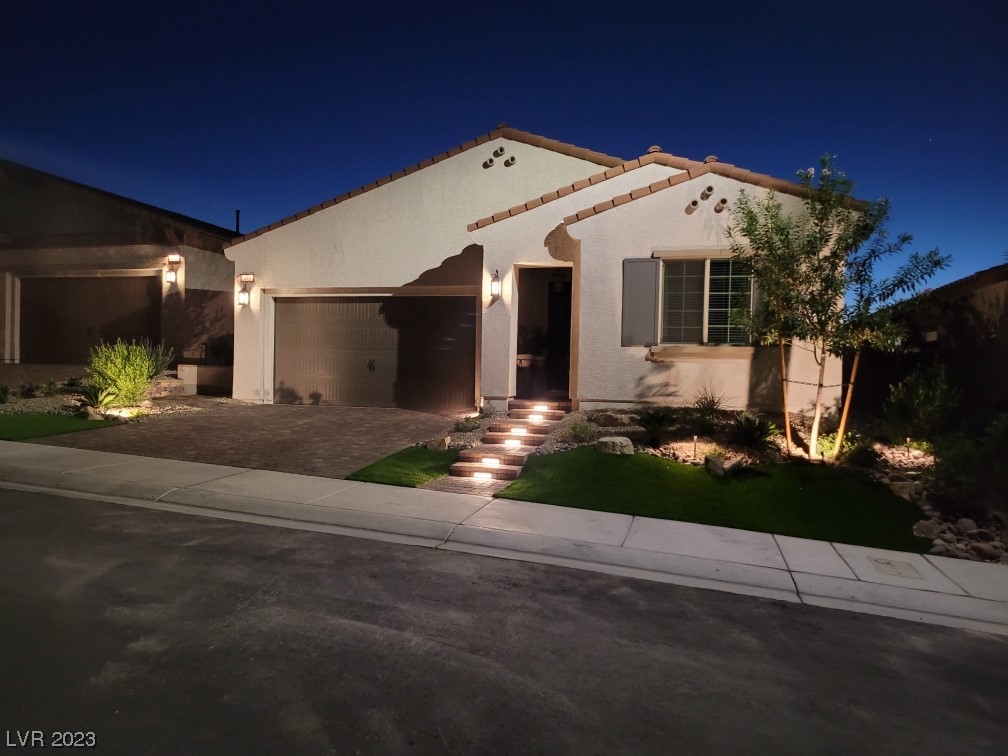The image showcases a small, well-maintained home that appears to be located in New Mexico, based on its architectural design. The sky is a dark blue, indicating that the sun has already set. The house features a white exterior with sections of light beige flat stone siding. It has three distinct roof tiers, each with light brown, clay-like shingles—one for the garage, one for the entryway, and likely one for the living room. The light brown garage door is situated to the left, accessed by a cement driveway. A set of lit stairs leads up to the front entrance, flanked by a neatly manicured garden with green grass and a small tree to the right. There's a single front window on the right side of the house. A light gray sidewalk runs in front, transitioning into a medium gray asphalt street. Flanking this home are houses on both the left and right. The overall scene captures a tranquil, suburban atmosphere just after dusk.